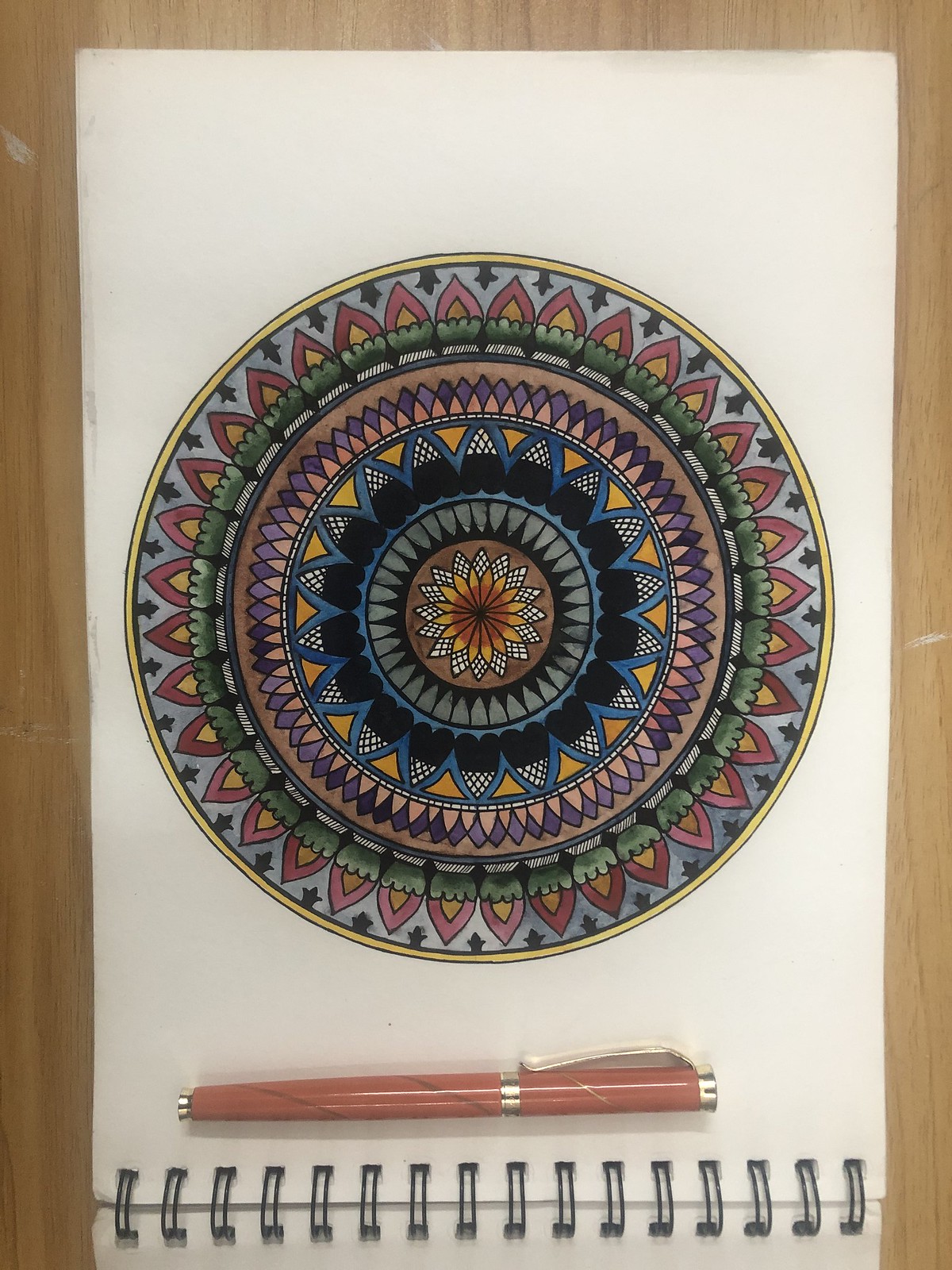This vibrant and intricately designed image features a series of concentric rings, each showcasing a distinct and abstract pattern. The outermost ring is adorned with a mesmerizing series of flame motifs, predominantly yellow at their cores and transitioning to red at their tips. Moving inward, the rings display a variety of shapes and colors, each differing significantly from the others in both hue and pattern. This creates a captivating, kaleidoscopic effect that draws the viewer's eye towards the center. At the bottom of the drawing pad holding this artwork, a pen can be seen, though its monochromatic appearance contrasts sharply with the vivid and complex artwork, suggesting it might not have been the primary tool used in its creation.